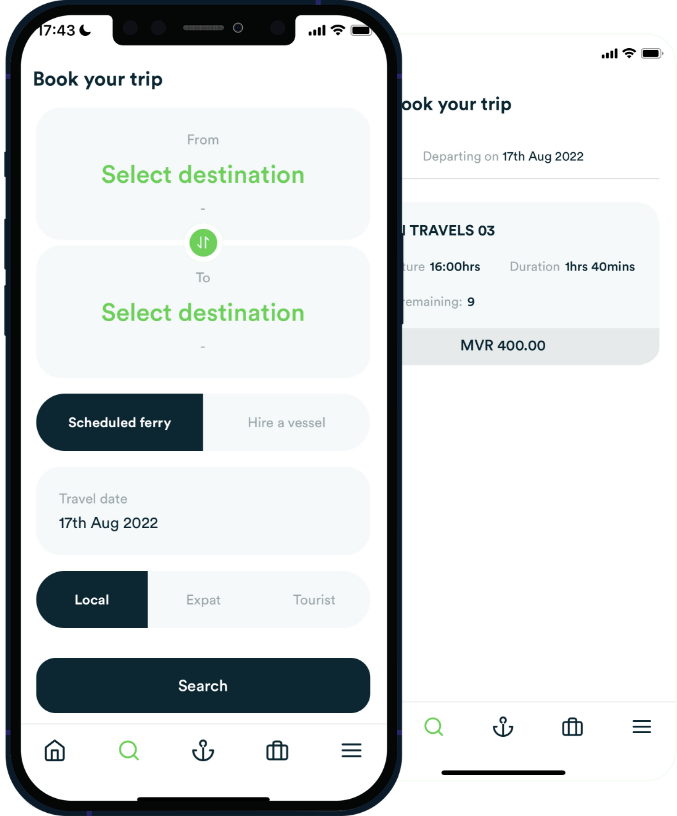The screenshot captures a mockup of a mobile application designed to facilitate travel bookings. The visual structure indicates it's likely a preview from a benefits section on a website, showcasing the app's features and functionalities.

On the left side of the image, a flat, front-facing illustration of a generic, black smartphone with rounded corners dominates the visual space. This mockup phone screen displays the app's interface, which appears quite detailed and colorful, rendered in a theme featuring light gray, green, and dark blue colors.

The interface highlighted within this mockup features several sections and options. At the top, instructions to "Book your trip" are displayed, presenting a form setup that includes 'From' and 'To' destination fields highlighted in green. Below this, two main action buttons, "Schedule Ferry" and "Hire a Vessel," are placed side by side, allowing users to choose one of the services.

Further down, there are selection options for traveler types, namely "Local," "Expat," and "Tourist," with "Local" currently selected. Above these options, it's noted that the travel date is set to "17th of August, 2022." Centered at the bottom of the mockup is a prominent "Search" button, designed with rounded corners in dark blue, featuring white text.

Additionally, the app's navigation menu is displayed at the very bottom of the screen. From left to right, it includes a dark blue "Home" icon, a green-highlighted "Search" magnifying glass icon, a dark blue "Anchor" icon, a "Suitcase" icon, and a "Hamburger menu" icon featuring three horizontal lines.

To the right of the mockup phone, there is partially visible information that extends out from behind the device. This information seems to be dynamically generated based on user inputs within the app. It includes travel details such as "Departing on 17th of August, 2022," with additional specifics like "Travels 03," "1600 hours," "Duration: 1 hour 40 minutes," and "Price: 9 MVR 400.00." However, parts of this text are obscured, adding a slight element of confusion.

At the top right corner of the screenshot, typical mobile device status icons are visible, indicating strong signal strength with four bars, a connected Wi-Fi signal, and a fully charged battery, providing additional context about the mobile environment.

This detailed simulation effectively demonstrates the app's user interface and the functionality it offers for travelers seeking to book transportation services.